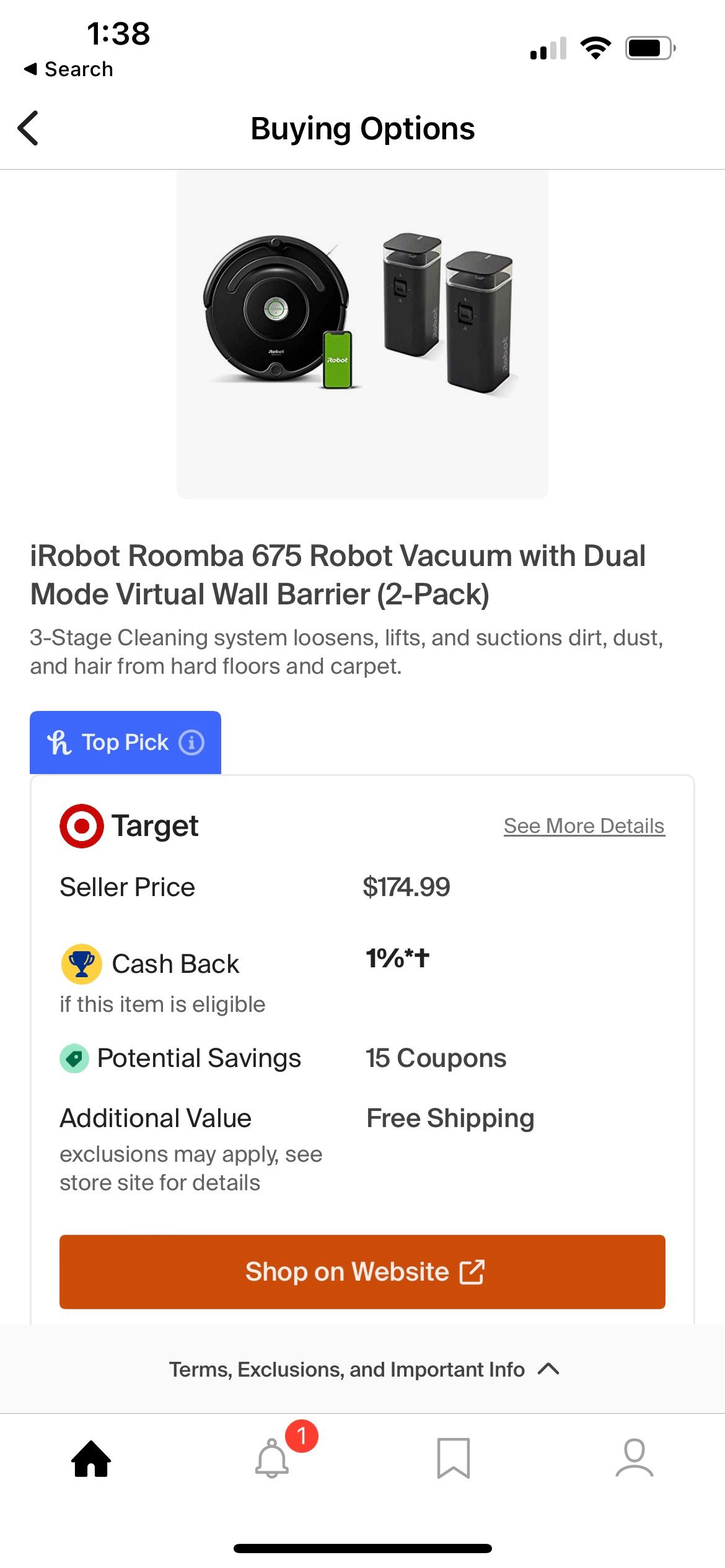In the image, a smartphone screen exhibits the Honey app being utilized to browse purchasing options for the iRobot Roomba 675 Robot Vacuum, packaged with a dual-mode virtual wall barrier in a two-pack listing. The time displayed on the phone is 1:38 PM, the device shows two bars of service out of four, full Wi-Fi connectivity, and a battery level at two-thirds capacity.

At the top of the screen, the Honey app displays a “Buying Options” header with a left-pointing arrow to navigate back. Directly below this header is an image showcasing the Roomba 675, a circular robotic vacuum cleaner. Adjacent to the Roomba vacuum, a smaller image of a smartphone screen showcases the Roomba app interface, and two virtual wall barriers are pictured on the right.

The item description beneath the Roomba's image, written in light gray text, details its three-stage cleaning system that efficiently loosens, lifts, and suctions dirt, dust, and hair from both hard floors and carpets. Below the item description, there is a blue button featuring the Honey logo and to its right, the text “Top Pick” accompanied by an information button.

The display continues with comparative pricing details, showing Target as a competitor with the Target logo preceding the name. The seller’s price is listed as $174.99. Additional benefits include 1% cashback if eligible, potential savings from 15 available coupons, and statements about additional value, exclusions, and free shipping.

An orange button with white text indicates "Shop on Website," followed by terms, exclusions, and important information. At the bottom of the screen, a navigation menu includes icons for the home screen, notifications (bell icon), bookmarks, and the user's profile.